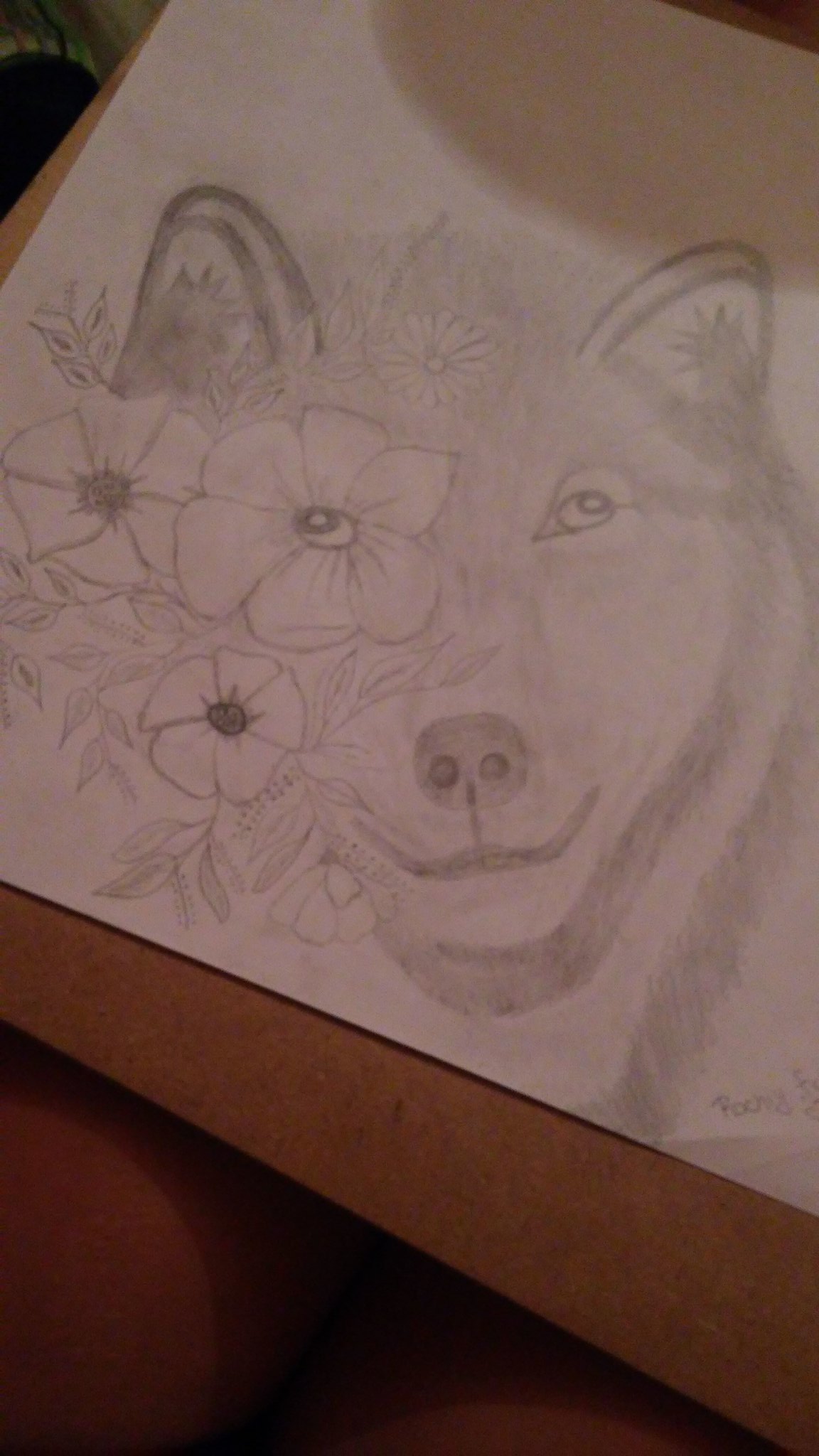The image showcases a meticulously drawn pencil illustration of a wolf’s face and neck. Dominating the composition is the wolf's striking visage, adorned with an array of intricately detailed flowers. A notable flower encircles one of its eyes, allowing the wolf’s eye to peer through it, adding a touch of mystique and allure to its gaze. Smaller floral patterns are delicately incorporated into its ears, and a tiny bloom is carefully positioned on its forehead. The artist has expertly depicted the texture of the wolf’s fur, particularly around the forehead and along the neck, giving the drawing a lifelike quality. The image includes the artist’s handwritten signature, signifying its authenticity. Presenting a balanced contrast between nature and wildlife, the drawing is set against a brown, square block background, which frames the artwork elegantly.